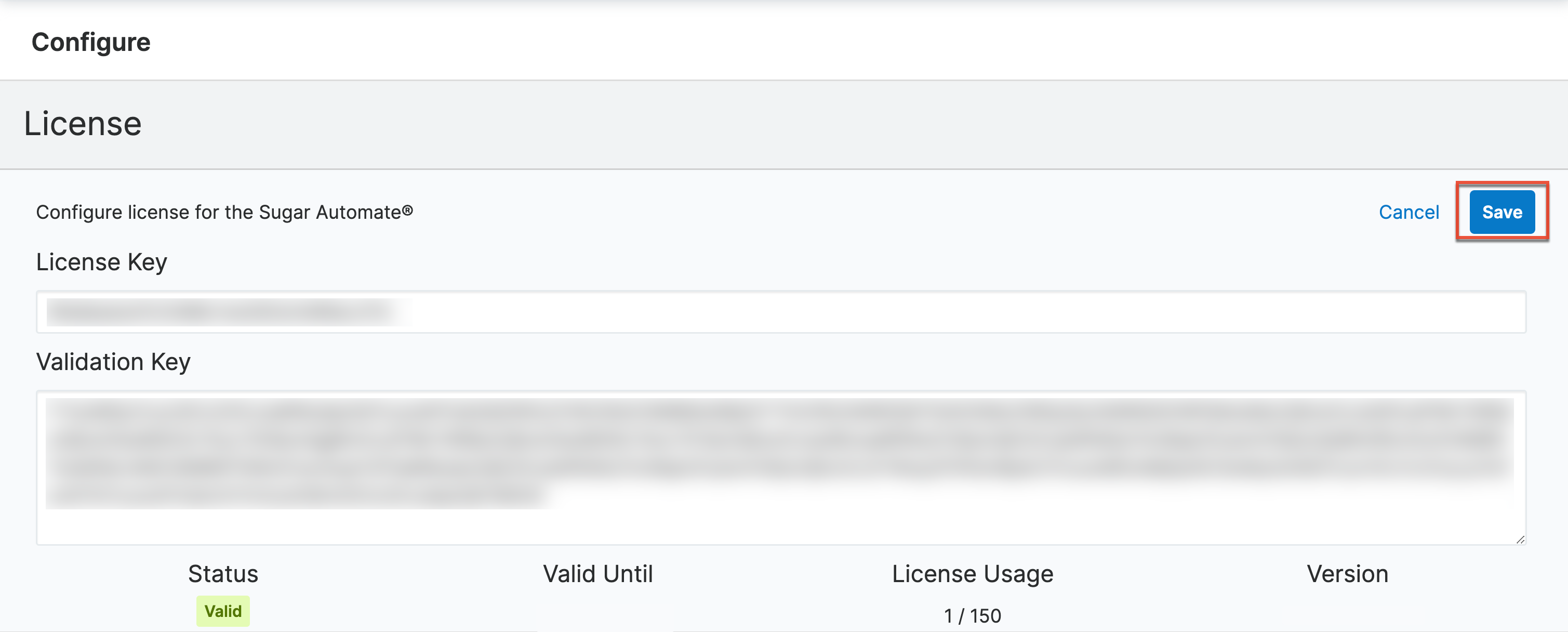The image features a website page with a white background and a thin gray border along the top. In the upper left corner, the word "Configure" is displayed. Below the top border, about an inch wide, is a light gray strip running down the left side, which has the word "License" written on it. Underneath "License," there's a section with a slight bluish tint. On the left side, in small letters, it reads "Configure License for Sugar Automate." Below this, in slightly larger text, it says "License Key."

On the right side of the page, there is a blue tab with the word "Save" written in white, and this tab is inside a red rectangle. To the left of the "Save" button, there is a blue "Cancel" button. 

Back on the left side of the page, there is a thin white bar that is about one-third filled with gray, with the remaining two-thirds being white. Directly beneath this bar, the text "Validation Key" appears in black font. Below this text is a large rectangle containing three horizontal lines that span the width of the rectangle, followed by another line that extends only about one-third of the way across. This shorter line is blacked out, obscuring whatever text or numbers might be underneath it.

Underneath this rectangle, there is a thin gray line. Moving back to the left side, about an inch from the edge, the word "Status" is displayed in black. Below this, in smaller lettering, it says "Valid." About two inches to the right of "Status," the text "Valid Until" is displayed in black. Another two inches to the right of this, the term "License Usage" appears, followed by "1/150" beneath it. On the far right side of the page, the word "Version" is shown in black text.